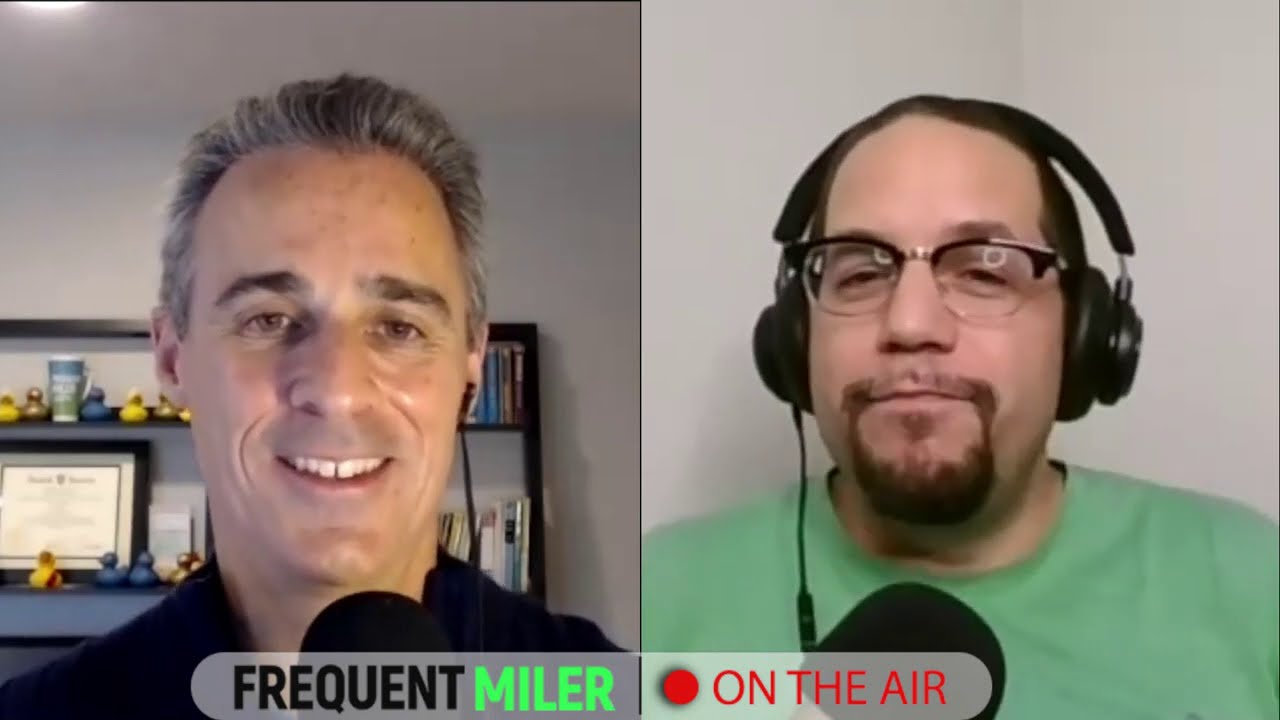In this split-screen image, reminiscent of a podcast interview, two men are engaged in conversation, each occupying one half of the screen. On the left side, depicted with a cheerful demeanor, is a man with olive skin and voluminous, grayish-black hair. He smiles broadly, showing his top teeth, and has a large, poofy microphone positioned at chin level. He wears a blue shirt, and behind him is a white wall with shadows cast on it. The background features a shelf holding a framed diploma, a cup, and various decorative items including blue and yellow rubber ducks, as well as some books on two visible shelves. The text "Frequent Miler" appears at the bottom of his screen segment, with "Frequent" in black and "Miler" in green.

On the right side is a lighter-skinned man wearing a green shirt. He dons black headphones with a wire hanging down and has a large, poofy microphone in front of him. His facial hair includes a mustache and a goatee, with closely shaved hair and a receding hairline. He also wears black-rimmed glasses with clear rims. The wall behind him is gray, providing a neutral backdrop. The text "On The Air" is displayed in a gray box at the bottom of his screen segment. The overall setup suggests they are engaged in a podcast or radio interview.